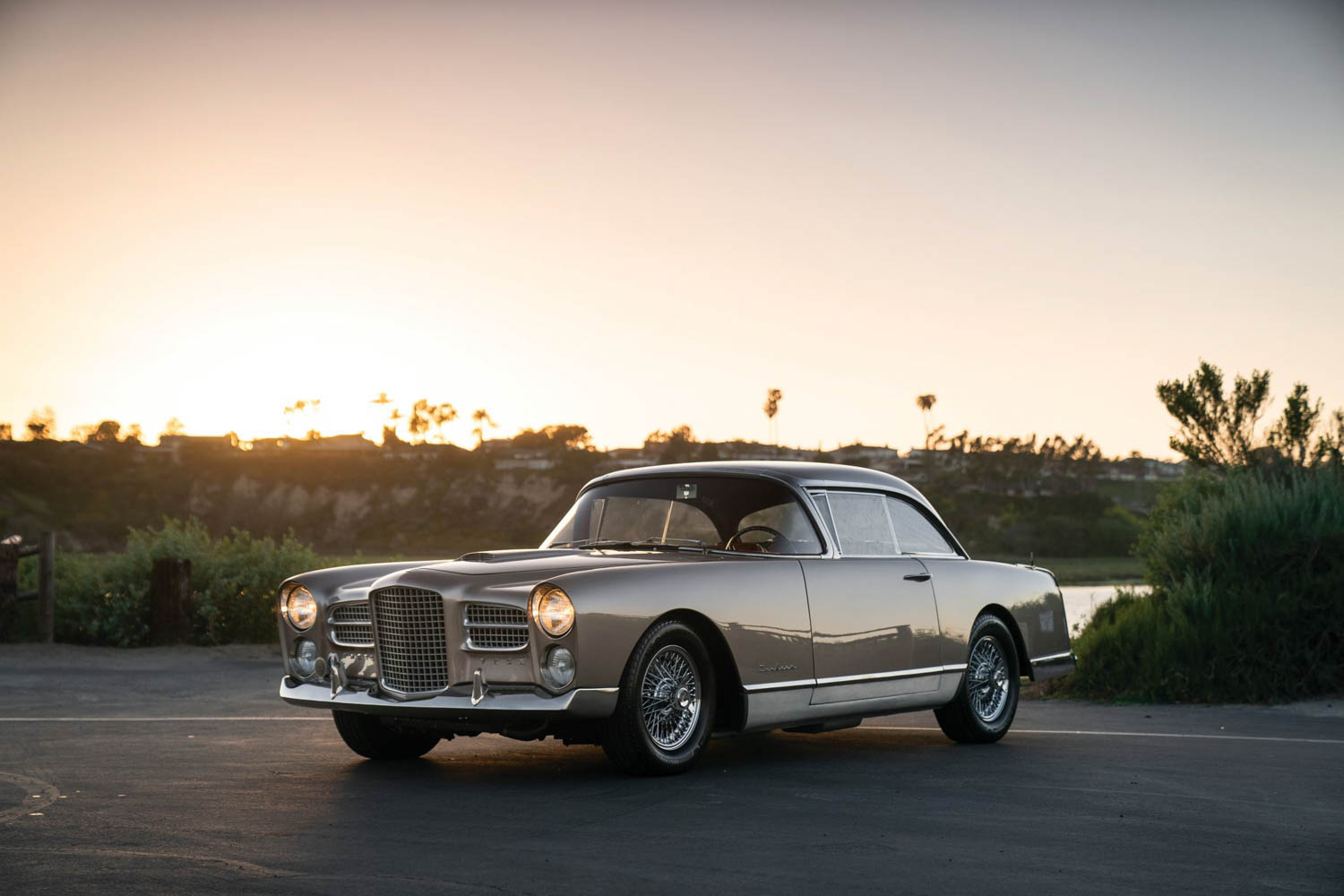The image captures a picturesque landscape scene featuring a stunning vintage two-door coupe-style car as its focal point. The car is parked on asphalt, highlighted prominently in the foreground. Boasting a unique taupe or beige exterior, which slightly morphs under the hues of the setting sun, the car's design elements include a wide front grille, two large round headlights that are illuminated, spoked tires, and a fully curved windshield. It is adorned with a large steering wheel indicative of its classic nature. Reflecting its surroundings on its polished surface, the car sits serenely as the golden hour paints the sky with brilliant sunset colors, devoid of clouds. In the background, a combination of natural elements includes sand dunes, a small waterway to the right, and scattered bushy greenery. Off to the left, distant silhouettes of buildings are faintly visible against the colorful horizon. The scene harmoniously blends the vintage elegance of the car with the tranquil beauty of the natural and semi-urban landscape.